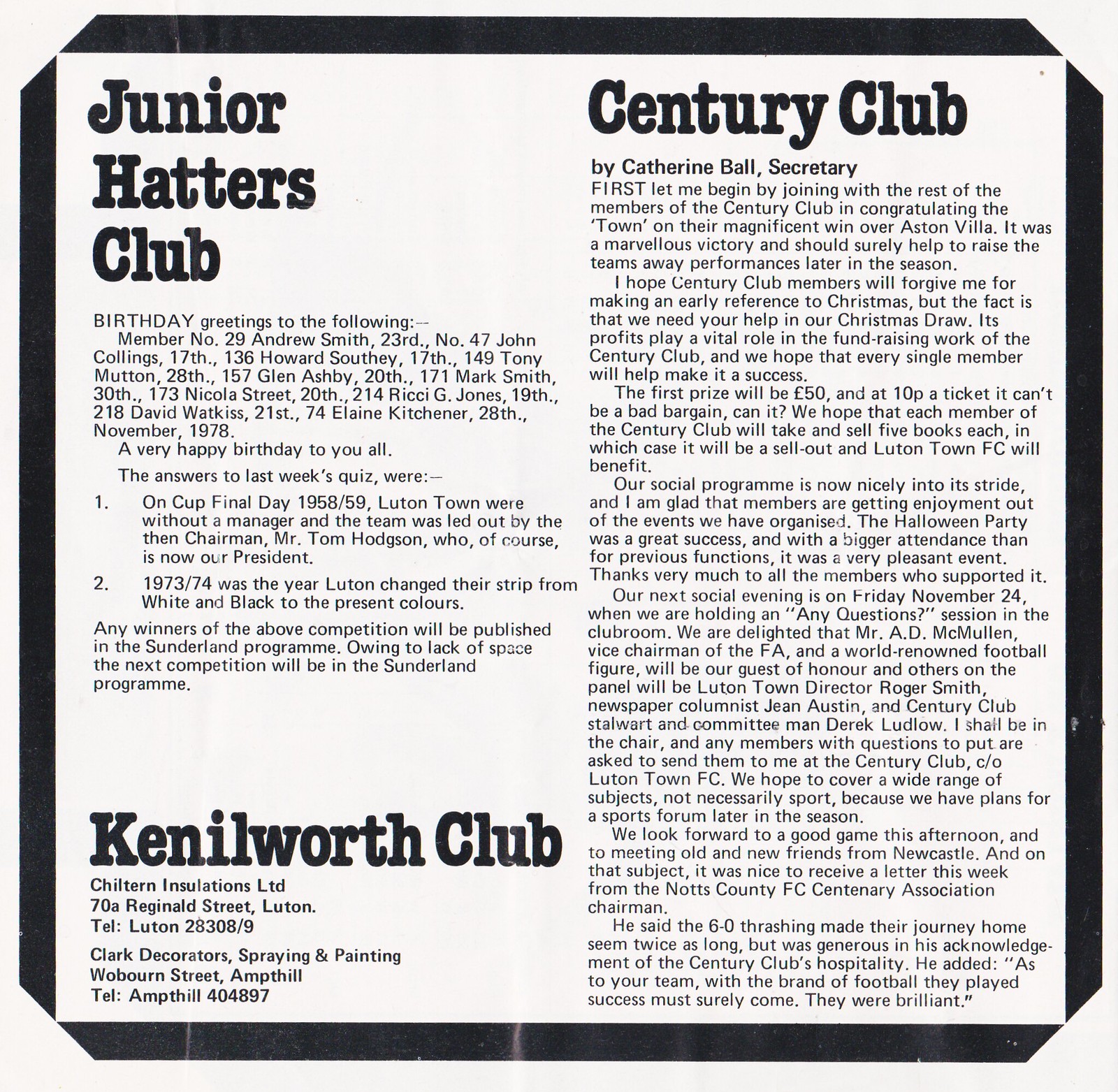The image is a scanned black-and-white page from what appears to be an old newspaper or magazine. The entire page is bordered with a thick black square, except at the four corners where the black border is cut off with white. The content is divided into two vertical columns.

In the left column, a bold black headline reads "Junior Hatters Club." Beneath this, there is a section titled "Birthday Greetings to the Following," listing members and their birthdays: number 29 Andrew Smith, 23rd; number 47 John Collings, 17th; 136 Howard Southey, 17th; 149 Tony Mutton, 28th; 157 Glenn Ashby, 20th; 171 Mark Smith, 30th; 173 Nicola Street, 20th; 214 Ricky G. Jones, 19th; 218 David Watkins, 21st; 74 Elaine Kitchener, 28th—all from November 1978. It then extends a happy birthday to all the mentioned members.

Further down, there's a section with the answers to last week's quiz: 1. On Final Cup Day, 1958-59, Luton Town were without a manager and were led by chairman Mr. Tom Hodgson, who is now the president. 2. In 1973-74, Luton changed their strip from white and black to the present colors. Any winners of this competition are to be announced in the Sunderland Program. Due to lack of space, the subsequent competition details will also be featured in the Sunderland Program.

At the bottom left, another bold black headline reads "Kenilworth Club," followed by advertisements for Chiltern Insulations Ltd., located at 70A Reginald Street, Luton (telephone Luton 28308/9), and Clark Decorators, specializing in spraying and painting, based in Woburn Street, Ampt Hill (telephone Ampt Hill 404897).

The right column is headed by "Century Club" in bold black print, authored by secretary Kathryn Ball. It begins with congratulations to the town for their win over Aston Villa, emphasizing the importance of the victory in boosting the team’s away performances. There's an appeal for help with the Christmas draw, essential for fundraising efforts, with a first prize of £50 and tickets priced at 10 pence each. Members are encouraged to distribute and sell five books each to ensure a sellout in favor of Luton Town FC.

The social program is noted as being successful, particularly highlighting the Halloween party. Upcoming events include an "Any Questions" session scheduled for Friday, November 24th, featuring Mr. A.D. McMullen (FA Vice-Chairman), Luton Town director Roger Smith, newspaper columnist Jean S. Austin, and Century Club committee man Derek Ludlow. Members are invited to submit their queries in advance.

The note closes by mentioning a letter from the Notts County FC Centenary Association chairman, who commended the Century Club's hospitality despite a 6-0 defeat, acknowledging the excellent performance and bright future of the Luton Town team.